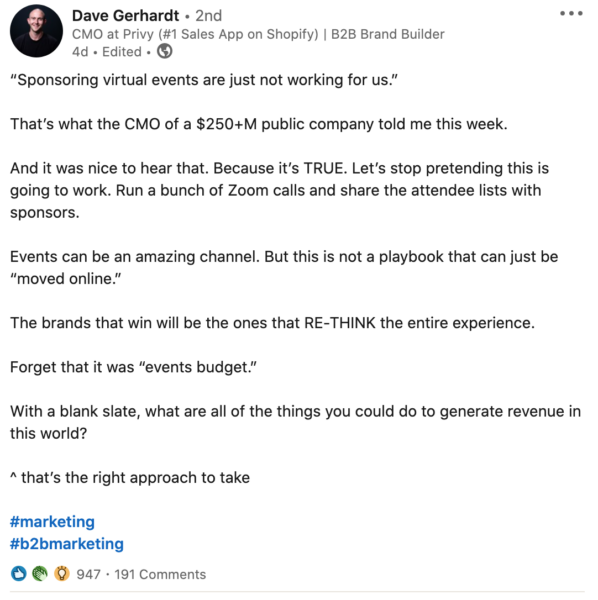Image Description: 

In this detailed caption for an image taken by Dave Gerhart, the text is divided into several informative sections:

1. **Profile Details**: 
   - **Image**: A professional profile picture of Dave Gerhart.
   - **Text**: 
     - "Dave Gerhart"
     - "CMO at Privy, number one sales app on Shopify"
     - "B2B brand builder"
     - "4D edited"
   
2. **Quote**: 
   - The quote by Dave Gerhart reads: 
     - "Sponsoring virtual events is just not working for us. This is what the CMO of a 250+ million public company told me this week, and it was reassuring to hear, because it's TRUE. Let's stop pretending this is going to work. Running a bunch of Zoom calls and sharing the attendees list with sponsors isn't effective. Events can be an amazing channel, but this is not a playbook that can just be moved online. The brands that WIN will be the ones that re-think the entire experience."
     - "With a blank slate events budget, consider all the things you could do to generate revenue in this world. That's the right approach to take."

3. **Hashtags**:
   - "#marketing"
   - "#B2Bmarketing"

This caption highlights a critique of the effectiveness of sponsoring virtual events and emphasizes the need for innovative thinking to create successful brand experiences.